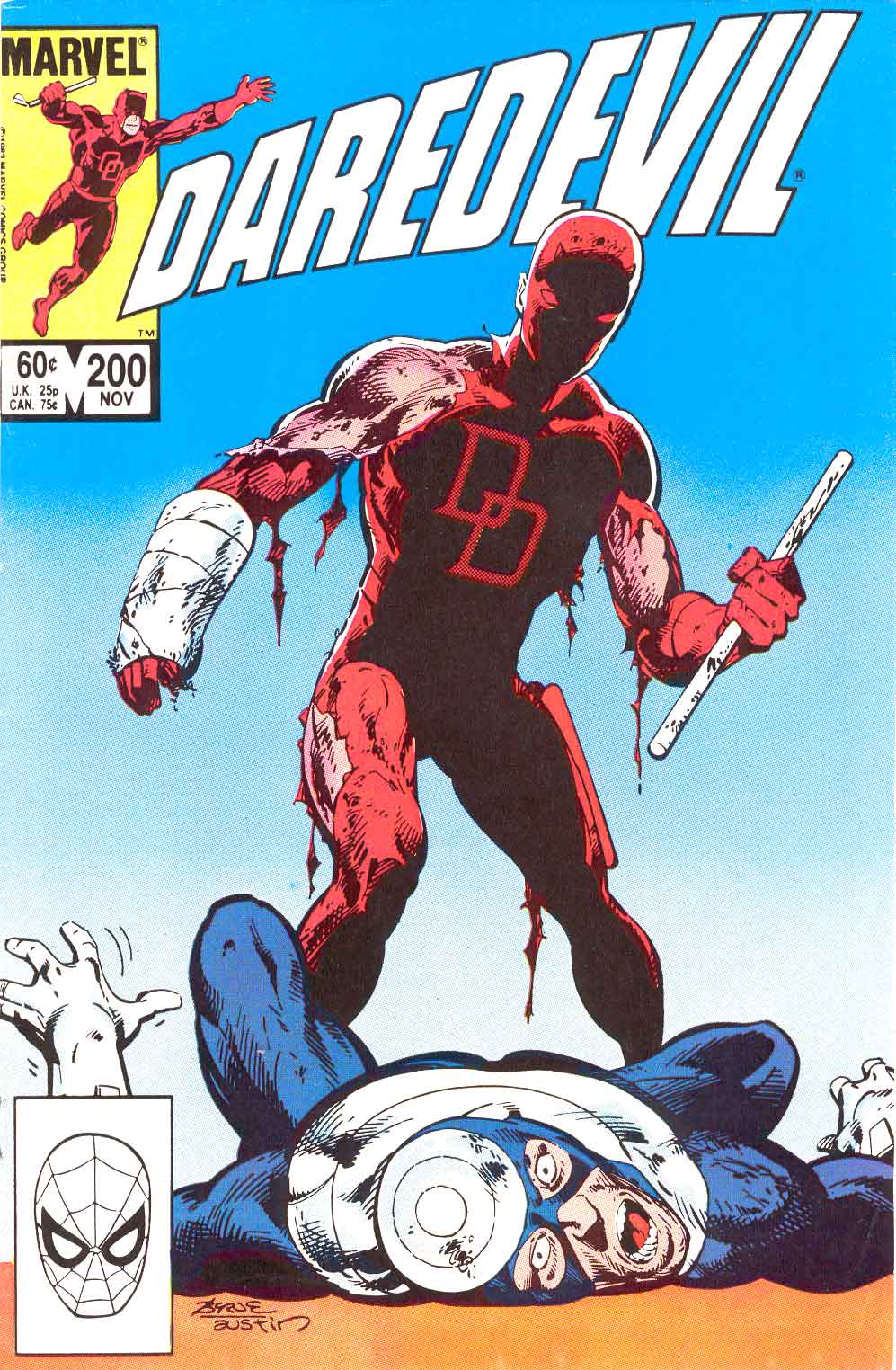The comic book cover is a detailed illustration of Marvel's Daredevil, Issue #200 from November. In the top left corner, there's a small yellow box with "Marvel" written in black, featuring a tiny figure of Daredevil in his standard red suit, appearing to leap forward. The price is listed as 60 cents for the US, 25 pence for the UK, and 75 cents for Canada. Dominating the cover is Daredevil himself, depicted in his iconic red costume, which is notably torn and tattered. His left arm has a cast, and he holds a white stick in his right hand. Daredevil stands over his opponent, Bullseye, who lies on the ground in a blue and white outfit, eyes widened, mouth agape, giving the impression of a fatal injury. The upper half of the cover is a spectrum of blues, transitioning to white towards the bottom, where a black and white pencil sketch of Spider-Man's face can be seen in the bottom left corner. The title "Daredevil" is prominently displayed across the top in bold white letters outlined in black. The comic has an artist’s signature near Spider-Man’s image, adding an authentic touch to this dramatic scene.